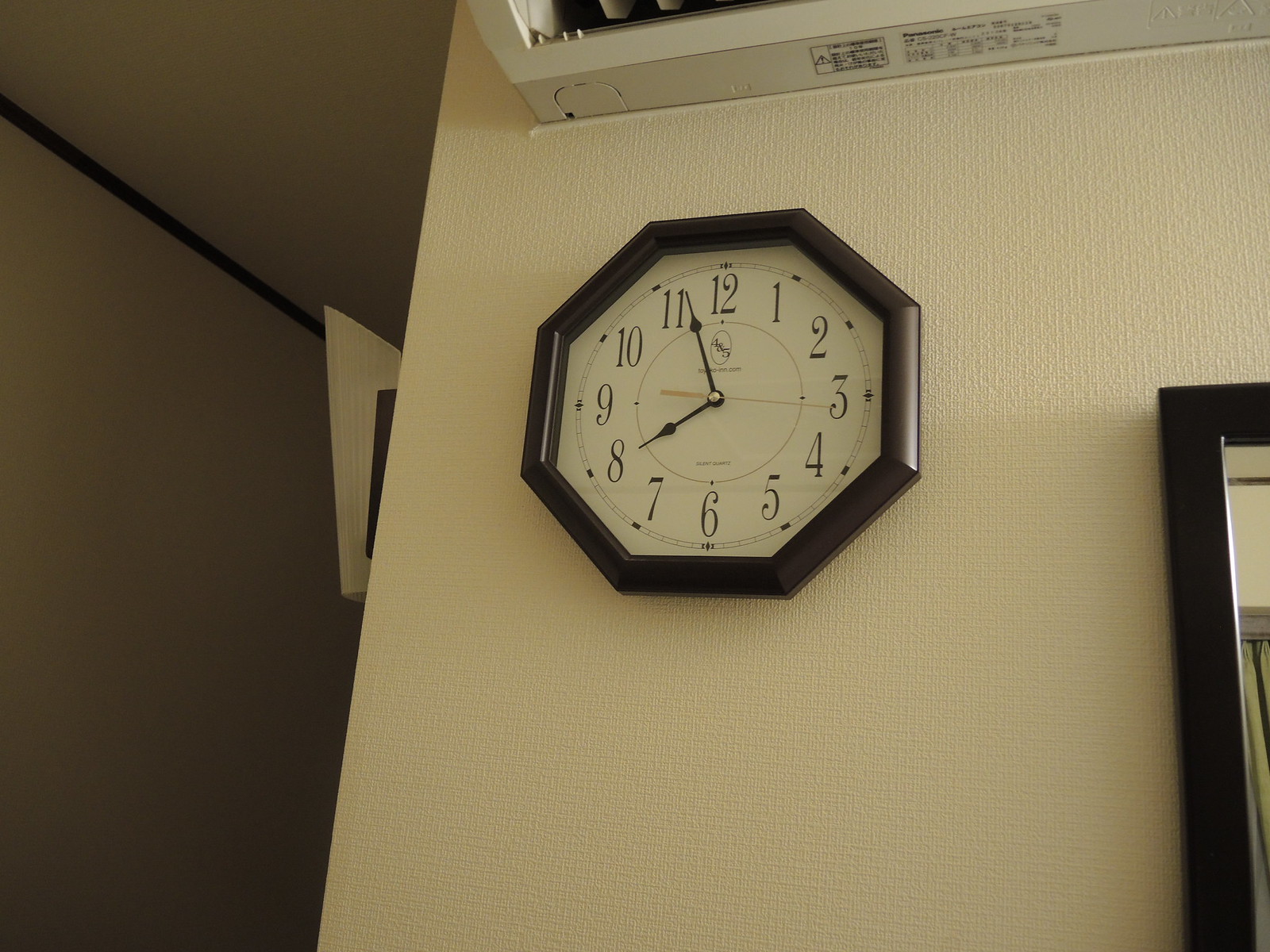The image captures an elegant octagonal clock mounted high on an exceptionally white, teal, or tan wall in a house. The clock, which has a dark wooden frame—either black or a rich dark brown—features two hands and is showing the time as 7:52. Positioned above the stylish clock is an air conditioning unit, while to the right, a partial view of a mirror can be seen, enhancing the room's aesthetic. The composition of the elements creates a balanced and sophisticated look within the living space.